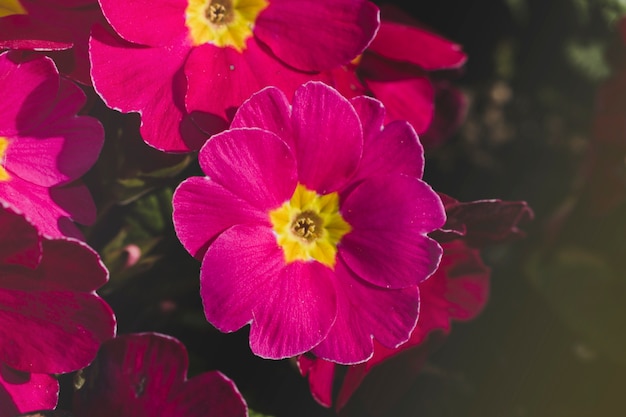This is a detailed close-up photograph showcasing vibrant purplish-pink flowers from a top-down perspective, with one prominently centered flower in full bloom. The petals are deeply colored, shaped uniquely with a two-piece appearance, resembling a round piece with a triangular cutout. These petals overlap in a circular arrangement around a distinct yellow center, forming a star or hexagon shape, with small fuzzy hairs visible. Surrounding this central flower are partial views of several similar blossoms, creating a sense of depth and abundance. The background is a mix of dark, blurry green and brown hues, suggesting leaves and bushes, enhancing the vivid colors of the flowers and emphasizing their striking beauty.